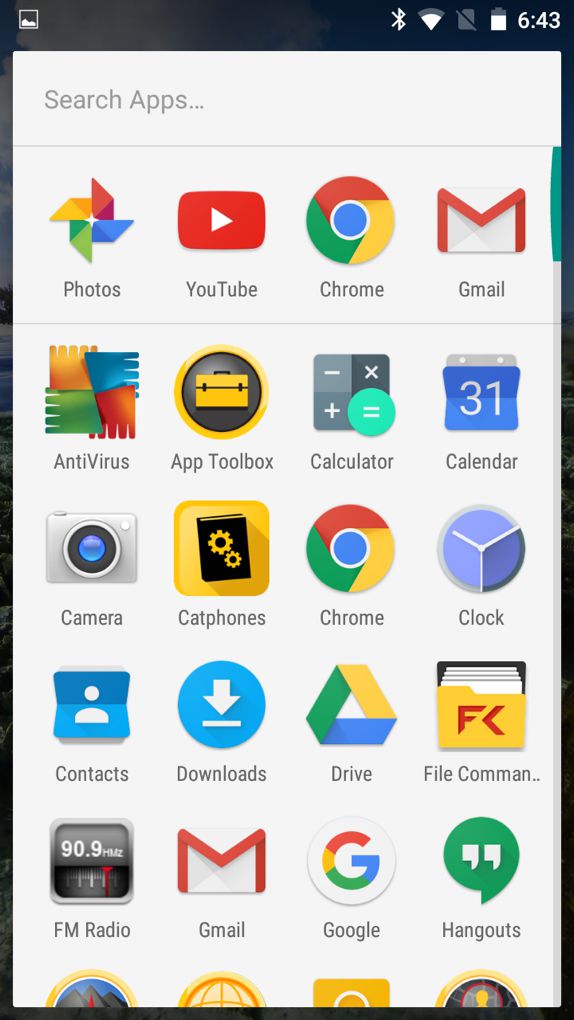This screenshot, taken from a mobile device, showcases the search menu used to locate various apps installed on the phone. At the top of the screen, the status bar displays important device information such as the current time, battery level, Bluetooth connectivity status, and Wi-Fi signal strength.

Directly beneath the status bar is the search menu, which allows users to search for specific apps. The displayed apps feature their respective icons and names for easy identification. In the first row, the visible apps include:

1. **Photos**: Represented by its distinctive logo.
2. **YouTube**: Identified by its red icon with a white play button.
3. **Chrome**: Marked by a circle divided into multiple colors representing the Google Chrome browser.
4. **Gmail**: Displayed with an icon of a white envelope bearing a bold, red 'M'.

Subsequent rows continue to showcase more apps, each accompanied by their unique symbols and names, ensuring users can quickly recognize and access the applications they need.